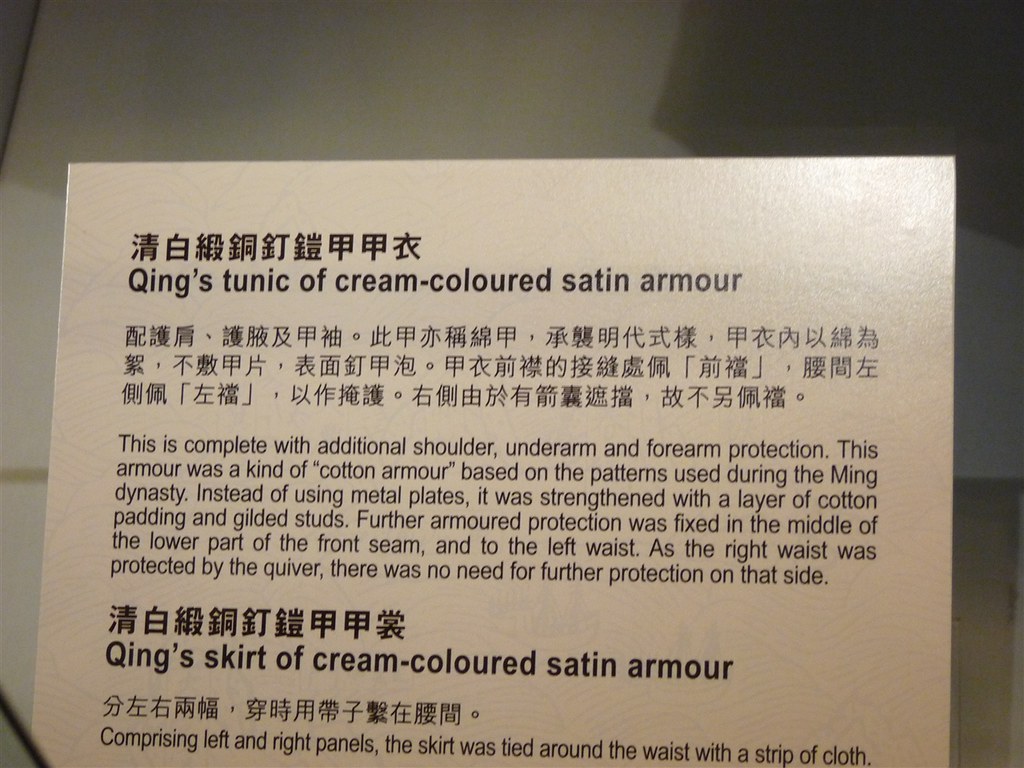This image features a detailed description presented on a white label with black lettering, accompanied by both Chinese and English text. The text begins with a line of Asian writing, followed by the English title: "Qin's Tunic of Cream-Colored Satin Armor." The description explains that this armor includes additional shoulder, underarm, and forearm protection. It was a type of cotton armor inspired by patterns from the Ming Dynasty, strengthened not with metal plates but with cotton padding and gilded studs. Extra armor protection was added to the middle of the lower part of the front seam and the left waist, while the right waist was sufficiently safeguarded by a quiver, negating the need for additional protection on that side. Further down, another line of Asian writing introduces "Qin's Skirt of Cream-Colored Satin Armor." This skirt, composed of left and right panels, was tied around the waist with a strip of cloth.